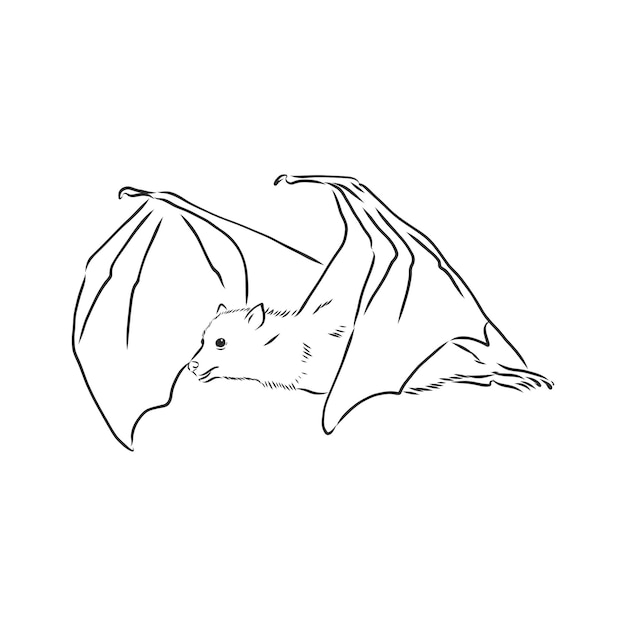The image depicts a simplistic black and white illustration of a bat in mid-flight, facing left. The bat's wings are arched upwards with distinct little hooks at their tips, creating a sense of motion. Its legs are stretched back along its horizontal, slightly tilted body, enhancing the impression of flight. Despite being mostly an outline, the bat features small, beady black eyes, tiny pointed ears, and a little mouse-like nose. There is subtle texturing to indicate fur on its head, neck, and legs, as well as detailing on its wings to show their curled, flapping nature. The bat's mouth is partially open, giving it an almost smiling expression. The overall drawing has a simple, perhaps crude quality, with no additional colors, set against a plain white background.